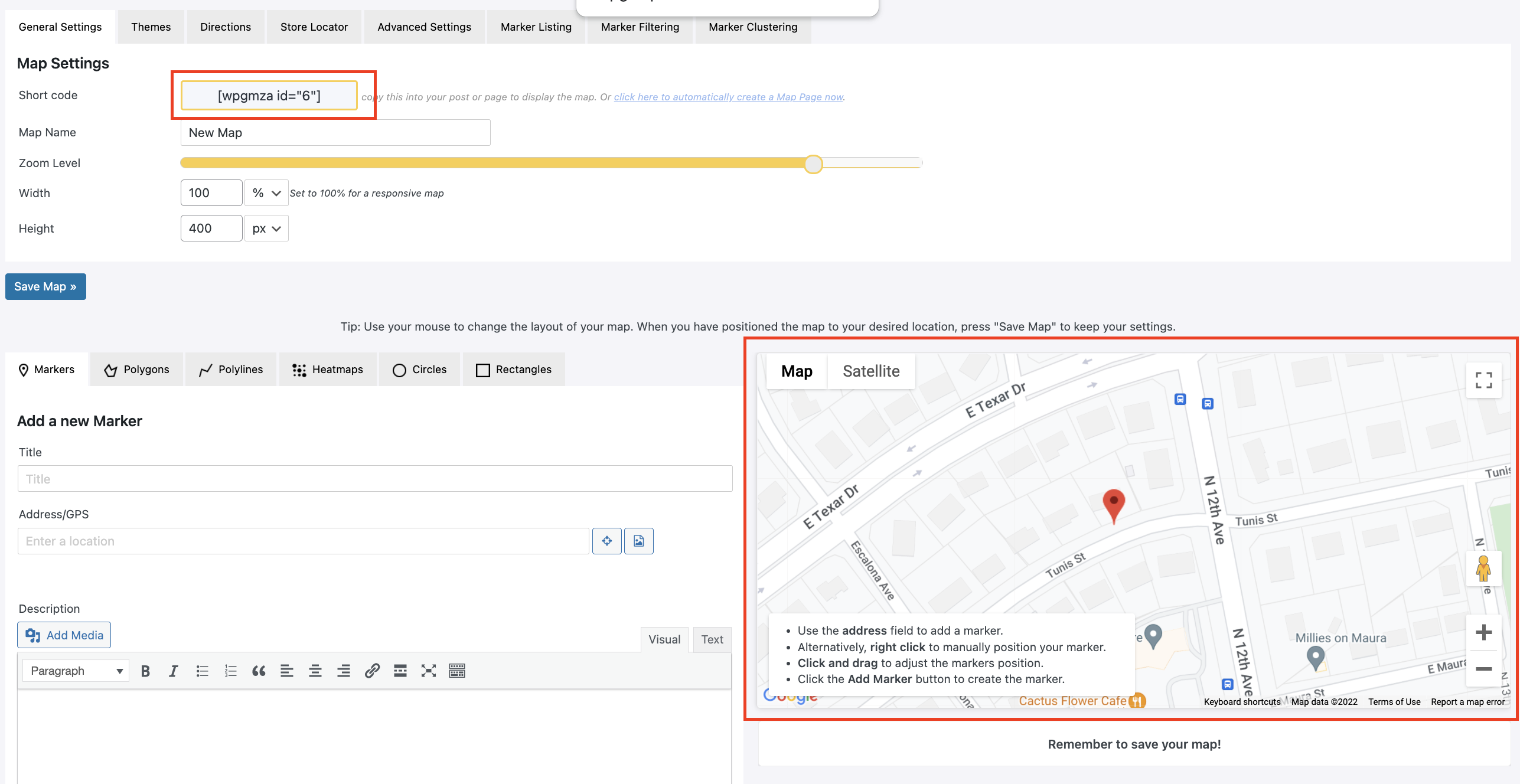The screenshot appears to be from a website interface featuring multiple tabs at the top for navigation. These tabs are labeled, albeit in small and difficult-to-read font, with categories such as "General Settings," "Themes," "Directions," "Store Locator," and "Advanced Settings." There is another tab possibly labeled "Listing," though it’s unreadable, as are the last three tabs due to their tiny font size.

Beneath the "General Listings" tab, prominently displayed in bold black font, is the heading "Map Settings." Below this are several sections, including some with small, unreadable text. Key interface elements include a yellow horizontal rectangle, framed by a red rectangle, followed by a horizontal yellow line filling roughly three-quarters of the width of the screen. This line starts about one-quarter of the way from the left edge and extends slightly beyond the center.

Below the yellow line, there are two dropdown fields stacked vertically. On the left edge of the image, a turquoise rectangular box containing white text (which is also hard to decipher) is centered vertically. The lower section of the interface features additional editable fields, dropdown menus, and an instruction in bold black font reading "Add a New Marker." Although the details in these fields are too small to discern, they appear to allow for customizable input.

To the right of the "Add a New Marker" section is a map with a red border. The map shows several streets and includes a red teardrop-shaped marker indicating a specific location. Text beneath the map provides a reminder to "Remember to Save Your Map."

Overall, the interface appears designed for customizable map settings, complete with multiple tabs for various features and settings that users can adjust.